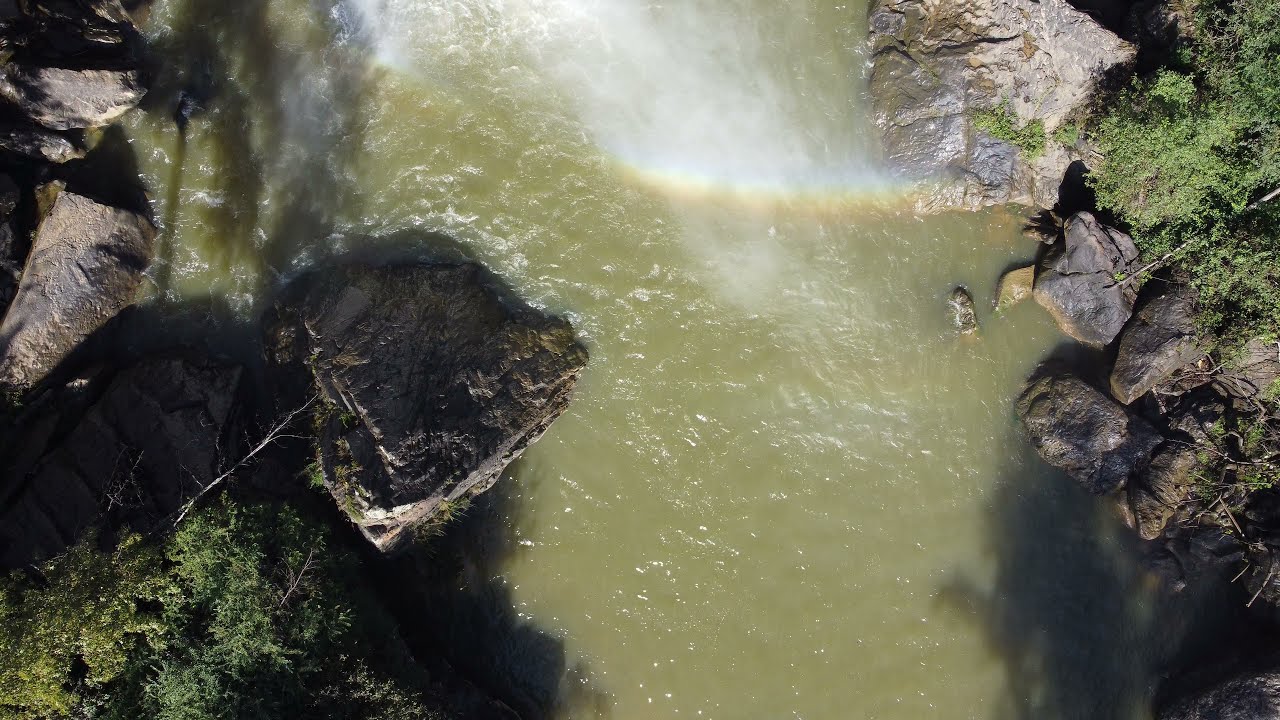The image presents an aerial view of a river rushing downwards, displaying a blend of dark green and tan hues in its waters. Set against a dramatic landscape, the river is bordered by large, scattered boulders and rocks forming the rugged shoreline. On the upper right side, a verdant tree stands tall, with lush green vegetation cascading over the boulders and rocks. Similarly, the bottom left corner showcases trees with green leaves and thick vegetation, though slightly above this area, dead trees lean ominously onto the rocks in the river's center. Adding to the image’s mystique, a multicolored rainbow arches from right to left near the top of the scene, created by the mist and water vapor rising from the river. The bottom right corner casts the shadow of a tree, extending across the river, emphasizing the river’s dynamic movement. The combination of overhead perspective and varied elements—boulders, tree shadows, mist, and rainbow—creates a striking and immersive natural tableau.